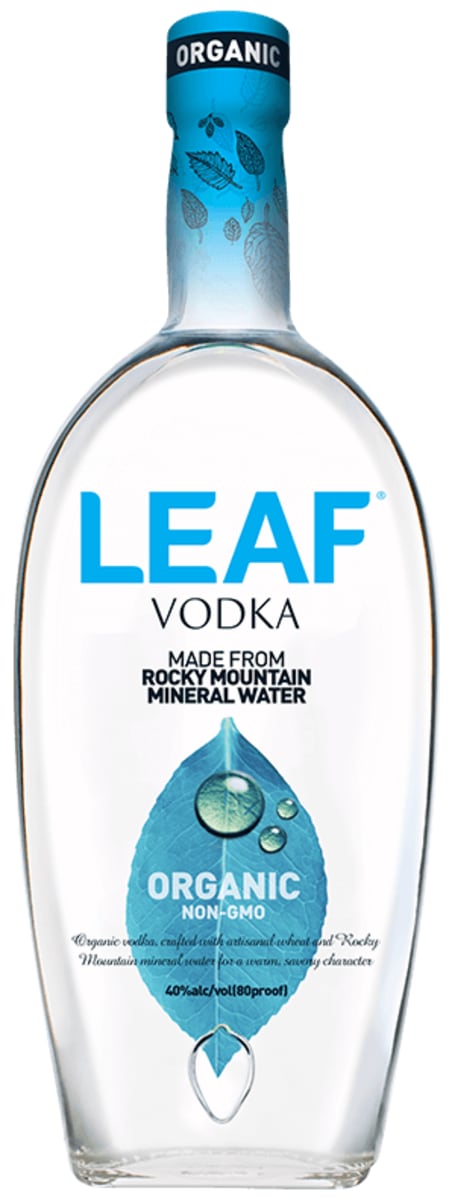This photograph features a bottle of Leaf Vodka displayed prominently against a plain white background. The bottle is crafted from clear glass with a slightly oval-shaped body, a flat bottom, and a glass stem. The neck of the bottle is adorned with penciled-in drawings of black leaves set against a blue background. At the very top, a black band with white text proclaims "Organic."

Descending the bottle, bold blue letters spell out "Leaf." Below this, in smaller black text, it states, "Vodka made from Rocky Mountain mineral water." Beneath this text is a prominent image of a blue leaf adorned with three droplets of water. White text on the leaf reads "Organic, Non-GMO." Further down, in fine script handwriting, it mentions, "Organic vodka crafted with artisanal wheat and Rocky Mountain mineral water for a warm, savory character." Below this, in bold black text, the alcohol content is specified: "40% Alcohol/Volume (80 Proof)."